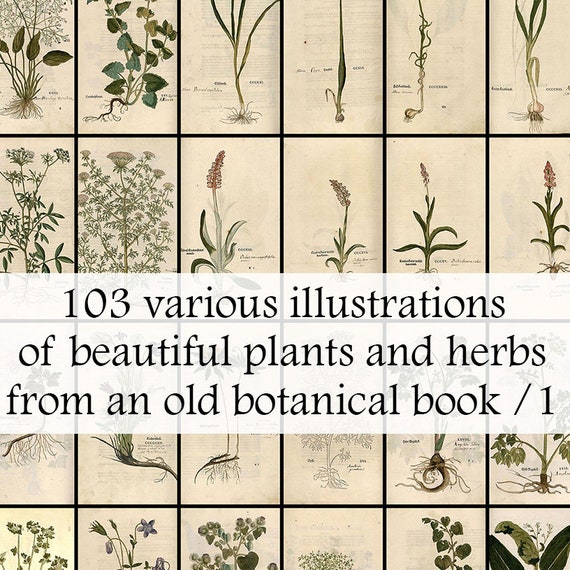This square image, approximately 4 inches by 4 inches, showcases a vintage botanical illustration collage with a total of 24 visible plant images arranged in a 6 by 4 grid, though the top and bottom rows are partially cut off. Each plant drawing is meticulously separated by thin black lines into distinct rectangular sections on a light tan or beige background. The plants are predominantly depicted in varying shades of green, some featuring flowers in hues of pink and cream, with intricate details extending from the roots to the stalks and buds. About two-thirds down the image, a transparent white banner spans horizontally, with three lines of black text that read, "103 various illustrations of beautiful plants and herbs from an old botanical book / number 1." The overall tone of the illustration is muted with dark green stems and leaves, some plants showcasing white bulbs and slender, diverse-sized leaves, contributing to its antiquated, serene aesthetic.